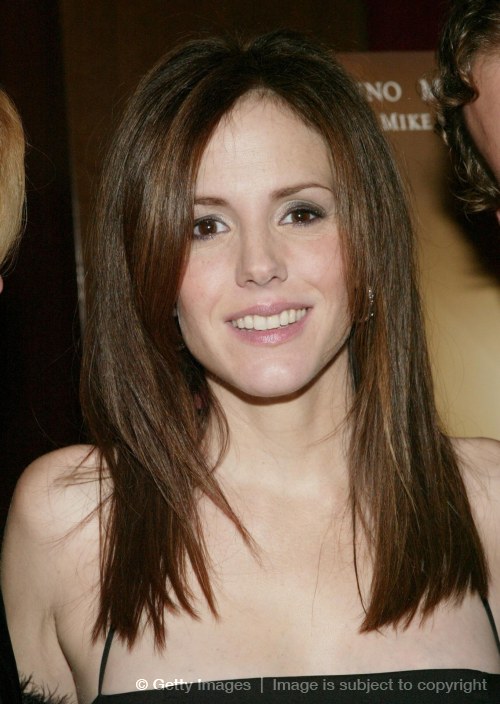The image captures a smiling woman who appears to be a celebrity, possibly an actress, with long hazel hair extending past her shoulders and hazel eyes. She is slender and dressed in a black outfit with thin shoulder straps, suggesting it might be a black dress. She is wearing silver or gold-tone earrings. The focus is on her upper body, making it difficult to identify the exact type of dress. To her left, there's a person with curly hair, but their face is not visible. The background features a dark banner with the word "Mike" partially visible. At the bottom of the photo, there's a watermark with "Getty Images" indicating the image's subject to copyright.